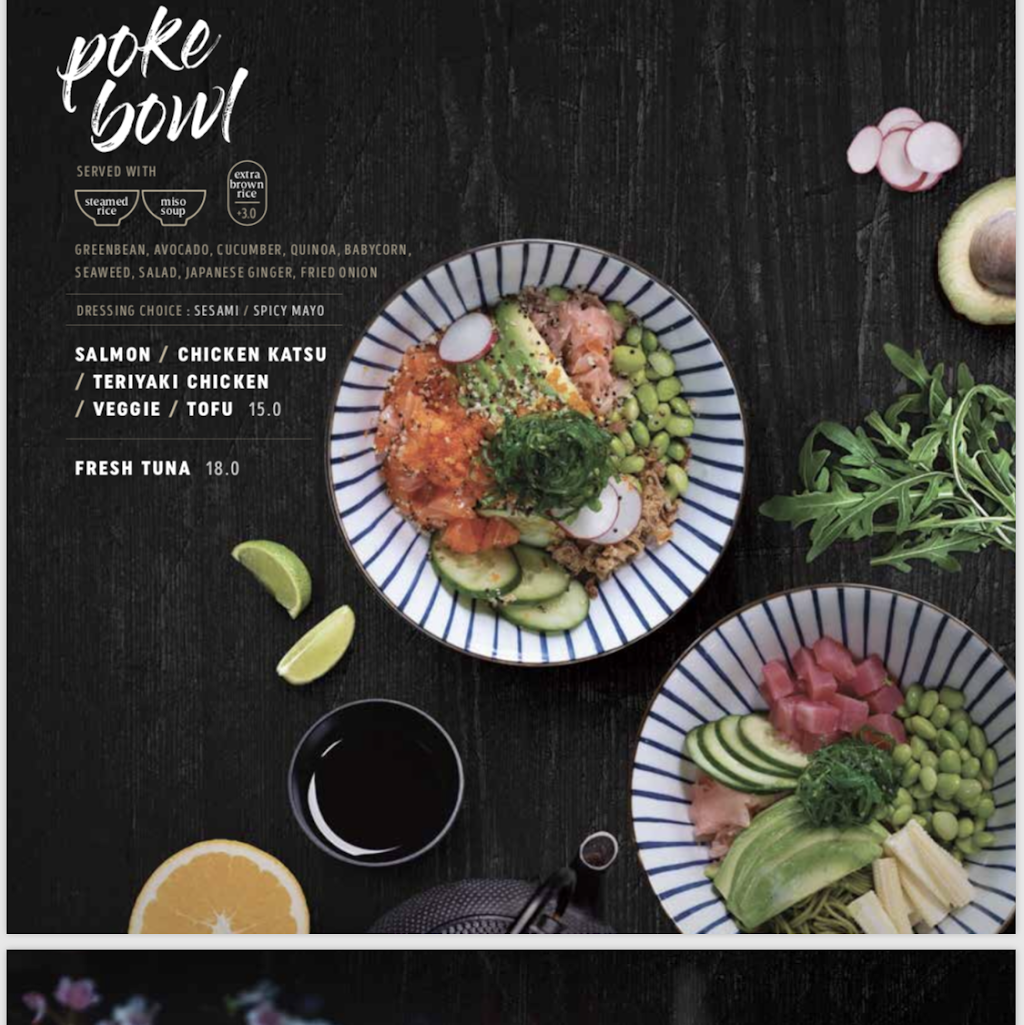The poster showcases a visually rich design with a background resembling a black-grained wooden table. At the top left corner, the name "Poki Bowl" is prominently displayed in white text. Directly beneath it, the phrase "Served With" appears in a light brown font, followed by a list of accompaniments: "Steamed Rice," "Miso Soup," and "Extra Brown Rice," each inscribed within light brown bowl-shaped icons.

Further down, additional serving options are detailed in light brown text, including "Green Bean," "Avocado," "Cucumber," "Quinoa," "Baby Corn," "Seaweed Salad," "Japanese Ginger," "Fried Onion," and "Dressing Choice:" with sub-options "Sesame" and "Spicy Mayo" highlighted in white.

Located in the middle left section, a white text menu lists protein options such as "Salmon," "Chicken Katsu," "Teriyaki Chicken," "Veggie," and "Tofu" priced at $15.00, while "Fresh Tuna" is marked at $18.00.

Central to the poster is a striking ceramic plate, predominantly white with blue outward lines near its edges. This plate features an appetizing assortment of ingredients including cucumber slices, various greens, avocado, red fish, green beans, and some sliced white vegetables.

On the bottom right, another similarly designed ceramic plate is showcased. This plate is garnished with cucumber slices, cubed tuna, green beans, sliced avocado, white vegetables, and a pale peach-colored meat.

The top right section of the table holds a pile of round, sliced vegetables, a halved avocado with its seed facing upward, and some green leaves. Meanwhile, the bottom left corner displays an orange slice, a small bowl of what appears to be soy sauce, and two slices of lime.

This meticulously crafted poster effectively highlights the diverse and vibrant offerings of the Poki Bowl restaurant.